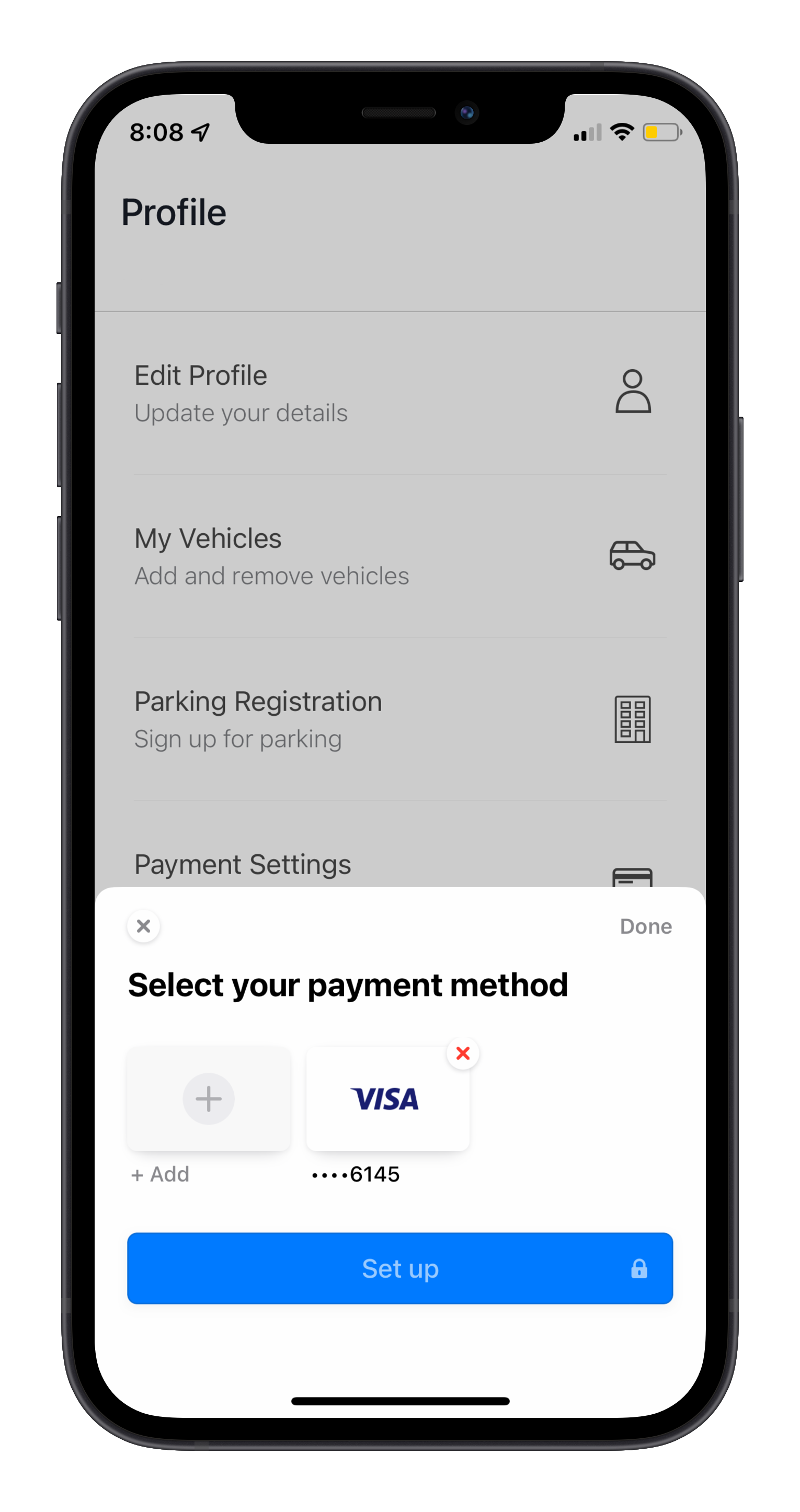A detailed image displayed on a smartphone showcases a payment method selection screen within an app. The phone features a thick black bezel with a prominent notch at the top, housing the time (8:08), a location arrow, service indicators showing 2 out of 4 bars, Wi-Fi connectivity, and a nearly depleted battery icon in yellow (15% or lower). The primary focus is the "Select Your Payment Methods" section, visible in a white box at the bottom of the screen. 

Users have the option to add a new payment method or select an already added one, such as a Visa card ending in 6145. The setup button for this card is highlighted with a blue bar. Behind this pop-up, the app's main interface can be partially seen, featuring different sections such as "Profile" (with options for editing profile and updating details, accompanied by an icon of a head and body), "My Vehicles" (allowing the addition or removal of vehicles, symbolized by a car icon), "Parking Registration" (indicated by a building icon, for signing up for parking), and "Payment Settings" (with a visible snippet of a debit or credit card icon).